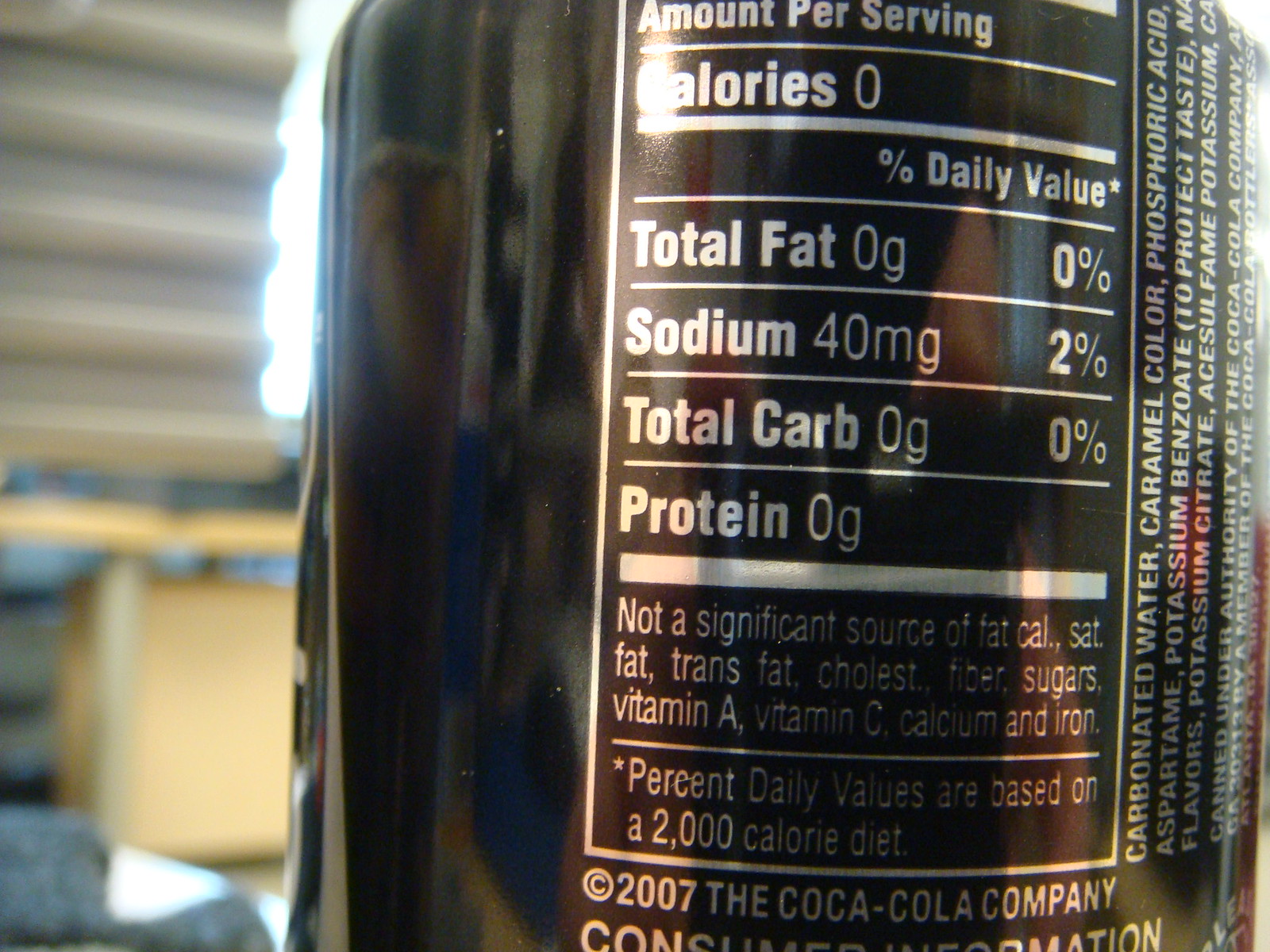This real-life photograph captures a close-up view of the back of a glossy black canned product, with a particular emphasis on the nutritional label adorned in a silver chrome color. The shiny surface of the can reflects the room it is in, though the recognizable hues from the reflection—natural wood tones, whites, and off-whites—do not clearly reveal the exact environment.

The nutritional label itself begins at the top with the heading "Amount Per Serving," followed by detailed nutritional information in descending order:

- **Calories:** 0
- **Total Fat:** 0 grams (0% Daily Value)
- **Sodium:** 40 milligrams (2% Daily Value)
- **Total Carbohydrates:** 0 grams (0% Daily Value)
- **Protein:** 0 grams

A thicker line separates this section from a subsequent note stating that the product is "Not a significant source of fat, cal, sat, fat, trans, fat, cholesterol, fiber, sugars, vitamin A, vitamin C, calcium, and iron." An additional line indicates that percent daily values are based on a 2,000-calorie diet.

Below this information, outside the silver rectangle, is a copyright symbol from 2007 attributed to the Coca-Cola Company. 

As the can curves to the right, the ingredients list comes into view, starting with "Carbonated water, caramel color, phosphoric acid," but the full content is obscured.

In the background, an out-of-focus interior setting is visible, featuring soft natural wood tones and off-white colors, contributing to a warm and familiar ambiance. Overall, the image directs attention primarily to the detailed nutritional and ingredient information printed on the can.